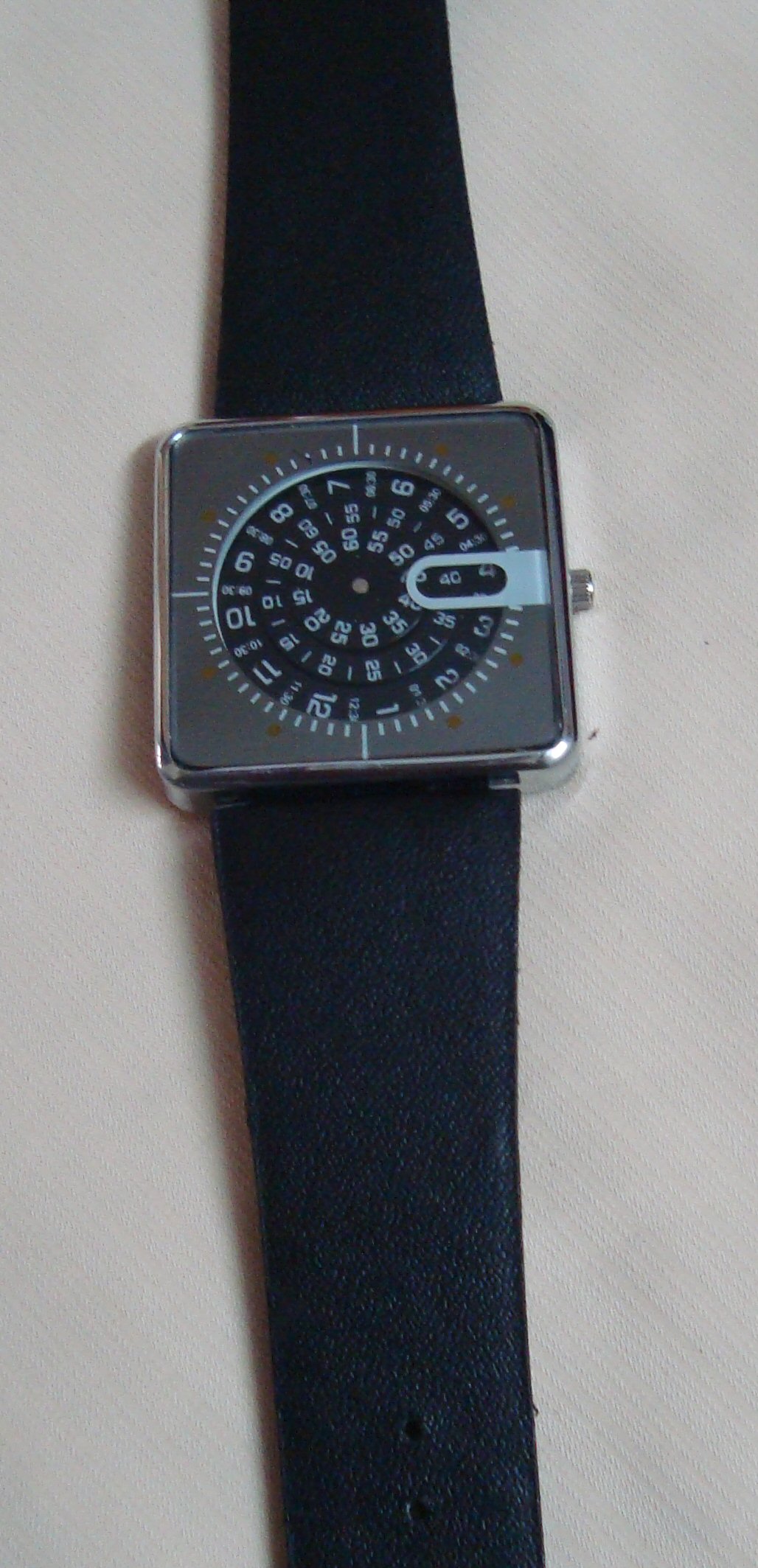Photograph of a unique watch placed on a flat white surface with subtle striations. The watch features a black leather band with a tapered design, wider near the square-shaped watch face. The watch face is unconventional, with a square outer frame but a circular area displaying the numbers. Multiple rings within the circular area display the time: the innermost ring starts at 5 and increases by 5s up to 60, the next ring also starts at 5 and ascends in 10s to 60 with smaller numerals, and the outermost ring showcases larger numbers from 1 to 12 alongside smaller, unreadable numbers.